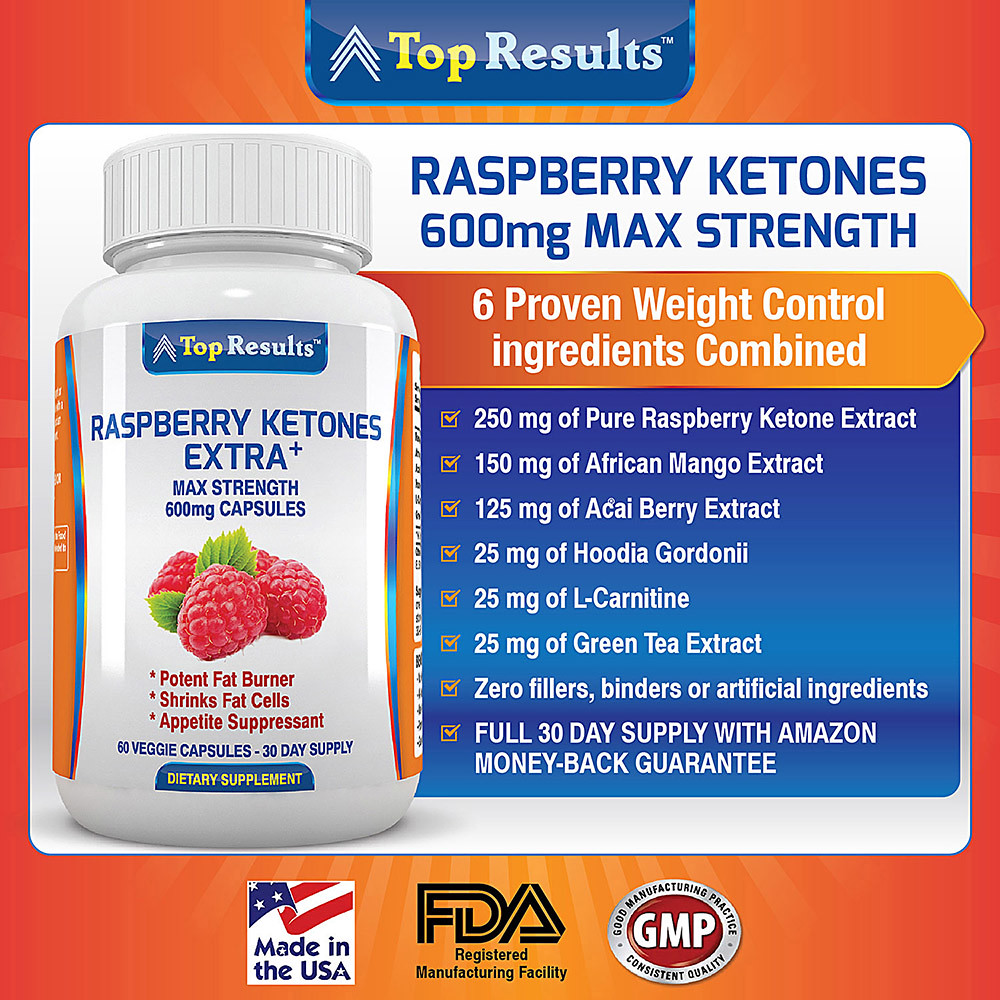The advertisement showcases a Top Results branded dietary supplement prominently featuring Raspberry Ketones Extra Strength. The product is contained in a bottle displayed on the left side of the ad, labeled with "Raspberry Ketones, Extra Strength, Max Strength, 600 mg capsules." The bottle also includes a realistic image of raspberries with green leaves. On the right side of the advertisement, a detailed list of the supplement's benefits and ingredients is presented, emphasizing its weight control attributes and potent fat-burning capabilities. Ingredients listed include 250 mg of pure raspberry ketone extract, 150 mg of African mango extract, 125 mg of acai berry extract, 25 mg of Hoodia gordonii, 25 mg of L-Carnitine, and 25 mg of green tea extract. The supplement boasts zero fillers, binders, or artificial ingredients and offers a full 30-day supply backed by an Amazon money-back guarantee. The ad features several endorsement stamps at the bottom, including "Made in the USA," "FDA Registered Manufacturing Facility," and "GMP Consistent Quality." The brand's name, "Top Results," is highlighted at the top in a distinctive yellow and white against a blue background. The overall advertisement background is a gradient of orange and red hues, adding a vibrant touch to the detailed presentation.